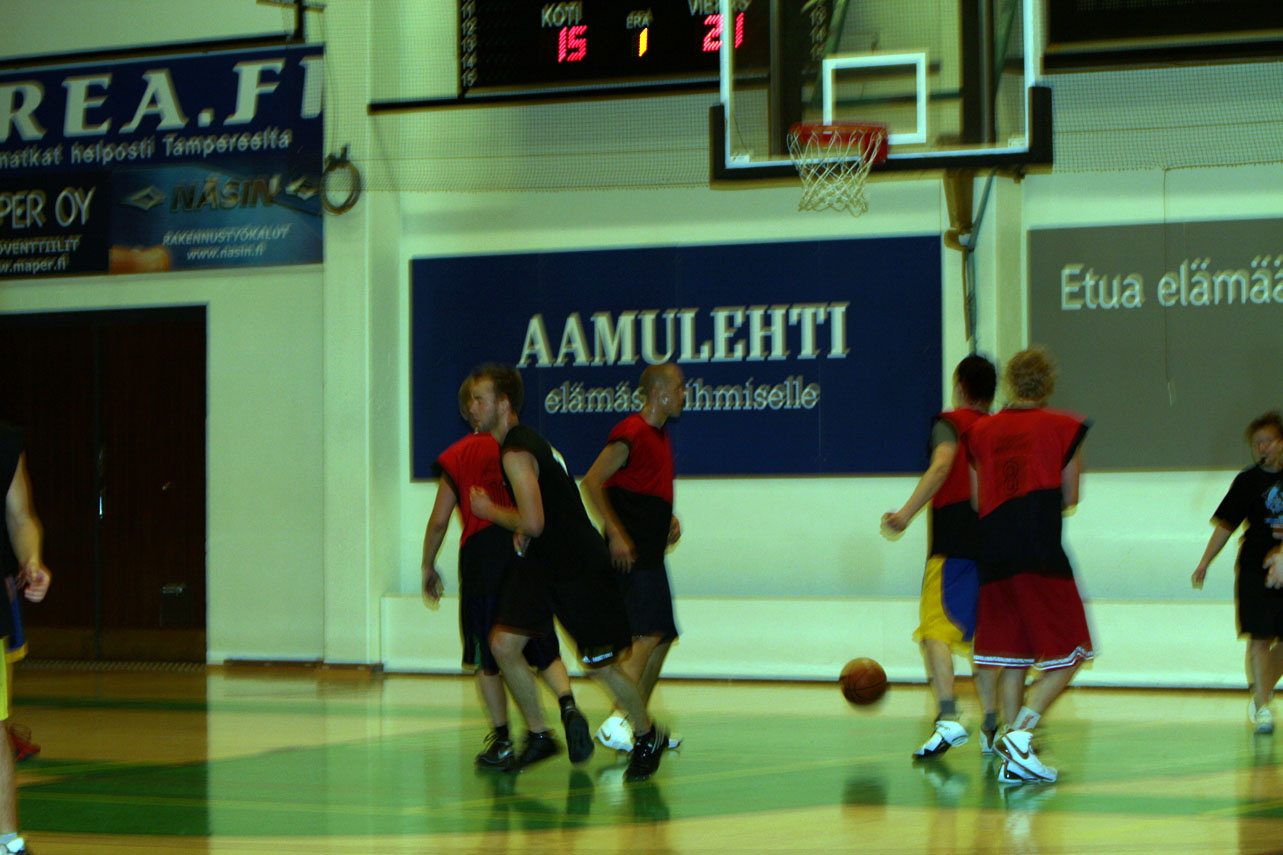This photograph captures an intense moment in what appears to be a high school or college basketball game. The players are energetically positioned on the court, dressed in their distinctive team uniforms. One team is clad in all-red tank tops paired with medium-length shorts, while the opposing team sports red shirts combined with black shorts. Adding a splash of color, a third individual is uniquely outfitted in a red short-sleeve shirt and striking yellow and blue shorts. 

On both sides of the court, spectators dressed in street clothes are visibly engaged in the action unfolding before them. The scoreboard, prominently displayed towards the top center of the image, features a black background with vivid red digits, displaying a score of 15 to 21. To the right and near the center of the photograph, a clear glass basketball hoop with a red rim and hanging net stands ready for the next shot. 

The gymnasium walls are adorned with numerous signs, written in a foreign language, enhancing the cultural context of the setting. These signs vary in color, with some being dark blue and one on the right side standing out in dark gray. The scene is a harmonious blend of athletic determination and the spirited atmosphere of a live basketball game.